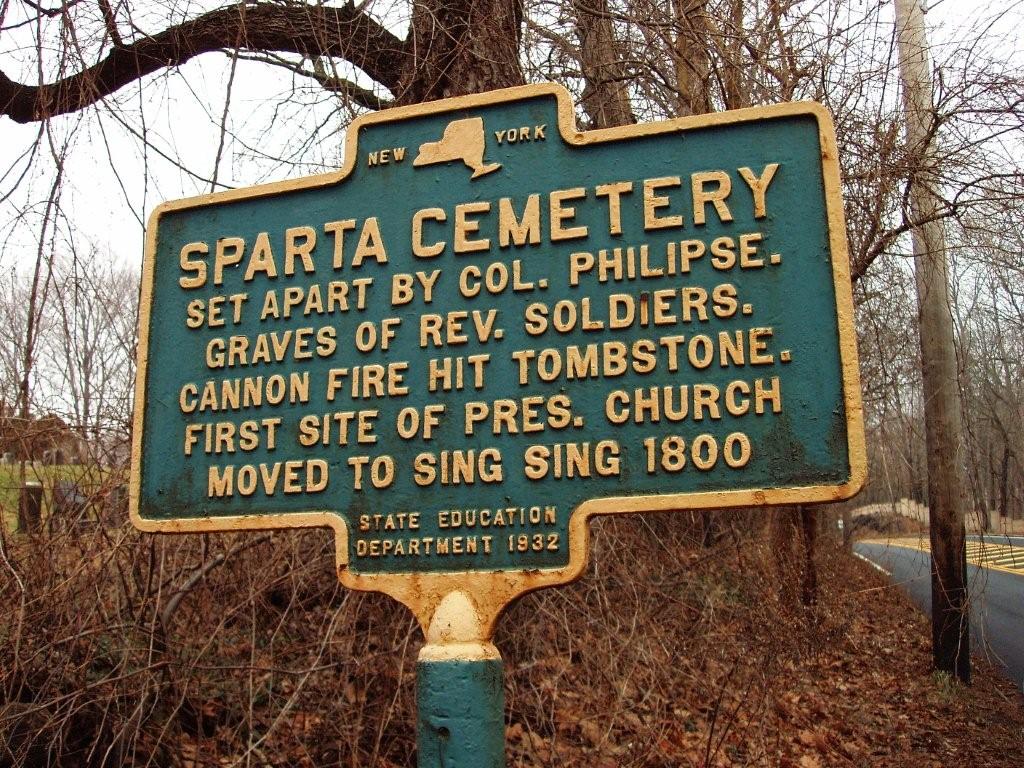The photo captures an old, weathered sign situated outdoors, depicting signs of age with rust spots and a dirty appearance. The sign is mounted on a green pole, with a thin gold border and a combination of green and teal hues inside. Positioned against a backdrop of dead-looking, brown woods indicative of fall, the rectangular sign's text is written in yellow.

At the top, the sign displays "New York" alongside an illustration of the state. Below, in smaller letters, it reads "Sparta Cemetery," followed by the phrase "Set apart by Col. Philips" and "Graves of Rev soldiers." Further down, it notes "Cannon fire hit tombstone" and mentions the "First site of Prez Church, moved to Sing Sing, 1900." At the bottom, in smaller text, the sign credits the "State Education Department, 1932."

To the right of the sign, there is a roadway visible, while on the left, part of a cemetery can be seen. The setting, combined with the fallen leaves and leafless trees, underscores the sign's historical significance and the passage of time.